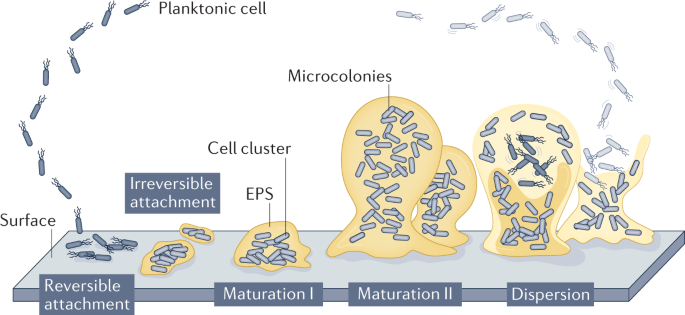The image is a detailed educational schematic from a science textbook, illustrating the life cycle of planktonic cells through various stages. The diagram uses a white background with shades of bluish-gray and yellow for clarity. From left to right, it showcases the following stages:

1. **Planktonic Cell**: The top left corner is labeled "planktonic cell," depicting small, cylindrical cells with tendrils.
2. **Reversible Attachment**: These cells are shown moving toward a blue-gray surface labeled "surface," where they temporarily attach.
3. **Irreversible Attachment**: Next, the cells are depicted clumping together and becoming encased in a yellow organic substance.
4. **Maturation 1**: This stage shows larger cell clusters labeled "cell cluster" and "EPS" (extracellular polymeric substances), indicating the initial phase of growth.
5. **Maturation 2**: The diagram illustrates the development into "microcolonies," where the clusters have almost tripled in size and start to grow vertically.
6. **Dispersion**: Finally, the mature clumps open up, releasing the planktonic cells back into the environment, ready to start the cycle again.

The overall color scheme—blue-gray and yellow—helps distinguish each stage clearly. This diagram effectively communicates the process of reversible and irreversible attachment, growth, and eventual dispersion of planktonic cells.